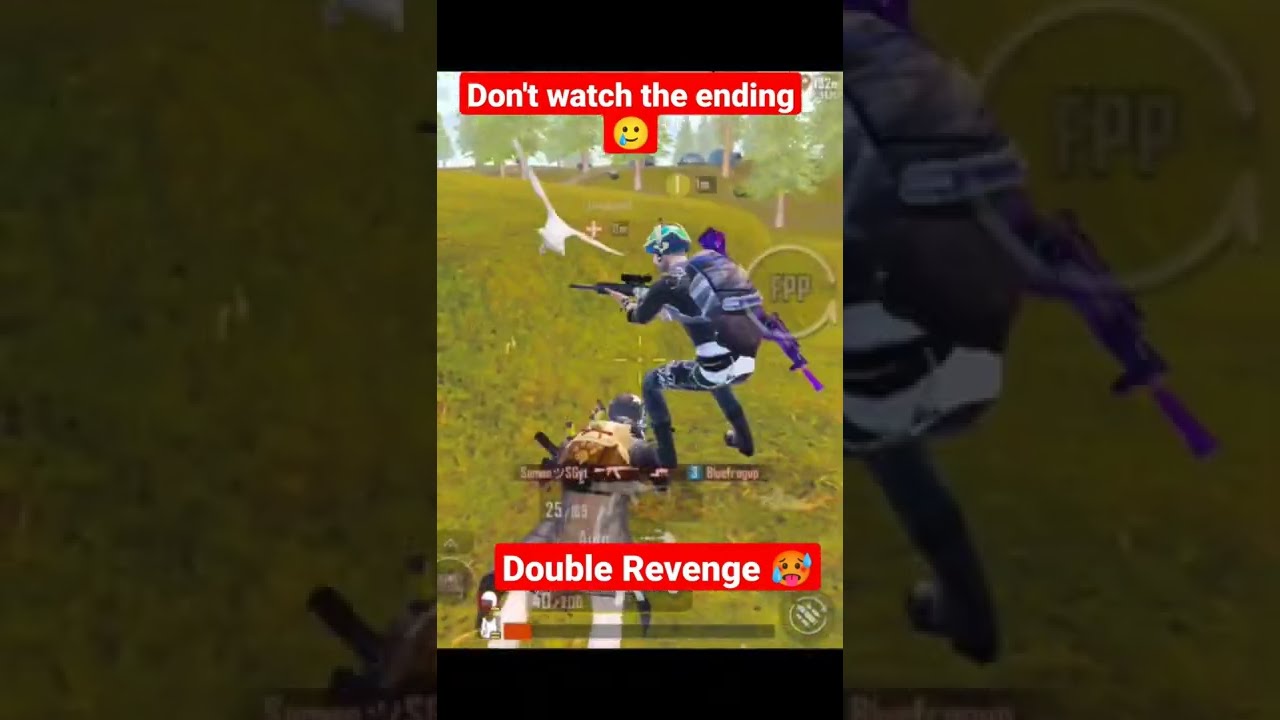A highly detailed vertical screenshot from a third-person shooter mobile video game is depicted. The image is divided into three distinct sections, with the left and right sides appearing darker, and the middle section being brighter. At the forefront, a video game character is crouched with a gun pointed to the left, while a second character is seen in a prone position, seemingly army-crawling on the grass, with their gun aimed at the crouched character. 

Both characters are equipped with rifles; the crouched character has a purple gun strapped to their back and a black sniper rifle in hand, wearing dark armor complemented by a teal-graded helmet. The crawling character lies with their back facing the viewer. A white bird is flying near the head of the crouched character. The background showcases a grassy field with sparse trees and distant buildings on a ridge line.

Overlaid on this scenery, the image features red text boxes with white writing: the upper banner reads "don't watch the ending," accompanied by a tearful smiley face emoji, while the lower banner states "double revenge," paired with an orange face emoji displaying tears and a protruding tongue. The central spot of the image has a crosshair marker, indicative of a shooter game interface.